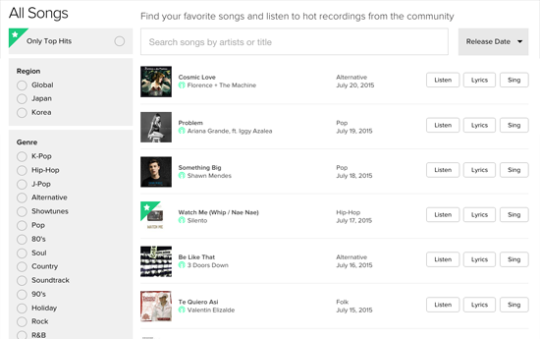The image is a screenshot taken from a computer or smartphone device, featuring a music streaming interface set against a white background, presumably the default background of the device. It includes a thin gray border at the top and on both sides. In the upper left corner, there is a label reading "All Songs" alongside a small green triangle with a white star inside it.

Below this area, within a gray box, the text "Only Top Hits" is displayed, followed by a small circle. Further down, there's a section labeled "Region" with three radio buttons labeled 'Global,' 'Japan,' and 'Korea,' none of which are selected. 

Proceeding to the "Genre" section, a variety of genre options are listed, including K-pop, Hip-hop, J-pop, Alternative, Show Tunes, Pop, 80s, Soul, Country, Soundtrack, 90s, Holiday, Rock, and R&B. Again, no genres have been selected.

At the top center, there's a motivational prompt: "Find your favorite songs and listen to hot recordings from the community." Below this, a search bar is available where users can search for songs by artist or title. Adjacent to this, there's a button labeled "Release Date."

The main area of the interface starts listing different songs, each accompanied by a small square image (likely album art), the song title, release date, and genre information. Additional buttons are present to listen to the lyrics, sing along, and perform other actions related to each song.